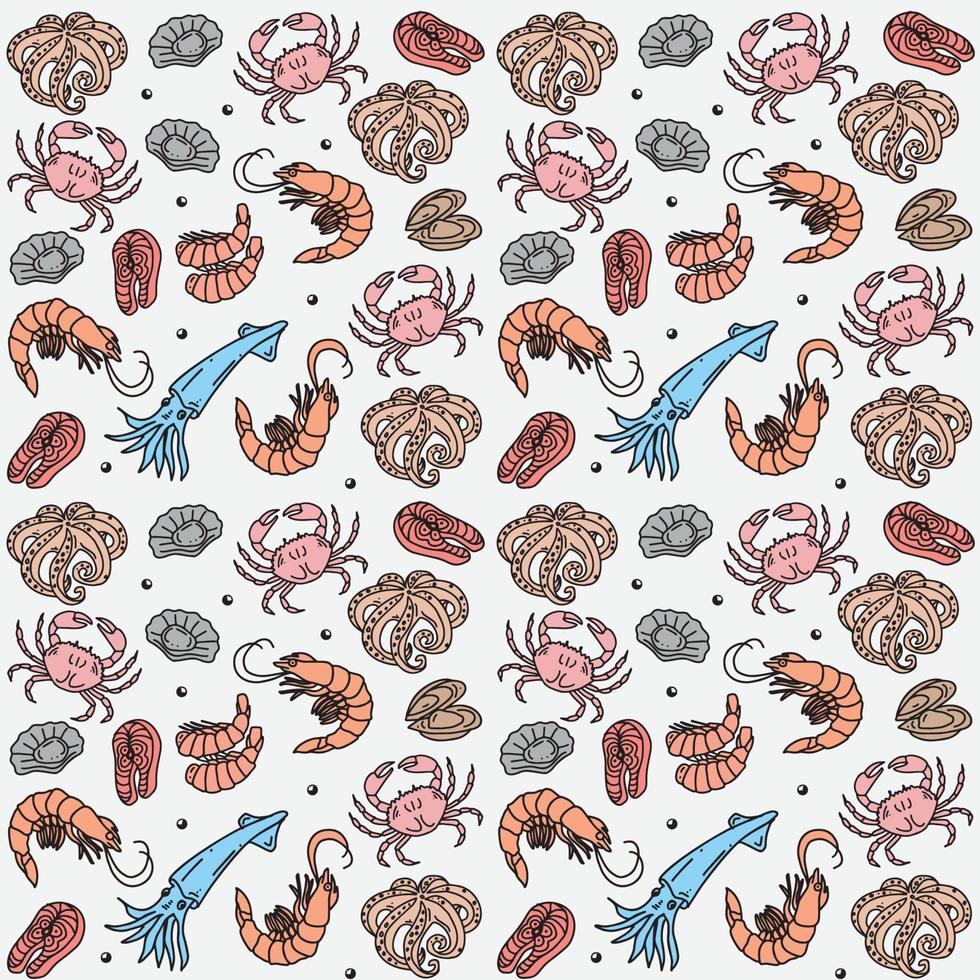The image depicts a whimsical, cartoon-like pattern of various sea creatures drawn in a repetitive and alternating fashion against a white background, resembling wrapping paper. The illustrations include a variety of marine life, such as a curled-up brown starfish with seven tendrils, a dark gray or black seashell, and an overhead view of a pink crab with its pincers almost touching above its head and legs flared out. Other creatures in the design include a clam, a mussel, multiple octopi, shrimp in different positions, a bay shrimp, a bluish squid, and intricate cross-sections of a pink salmon fillet. The sea creatures are colored in muted shades of pink, light salmon, light blue, gray, and reddish-pink. Small dots are interspersed between some of the illustrations, adding to the decorative nature of the pattern. The overall effect is a lively and repeating design, filling several rows and maintaining a consistent rhythm of motifs throughout the image.